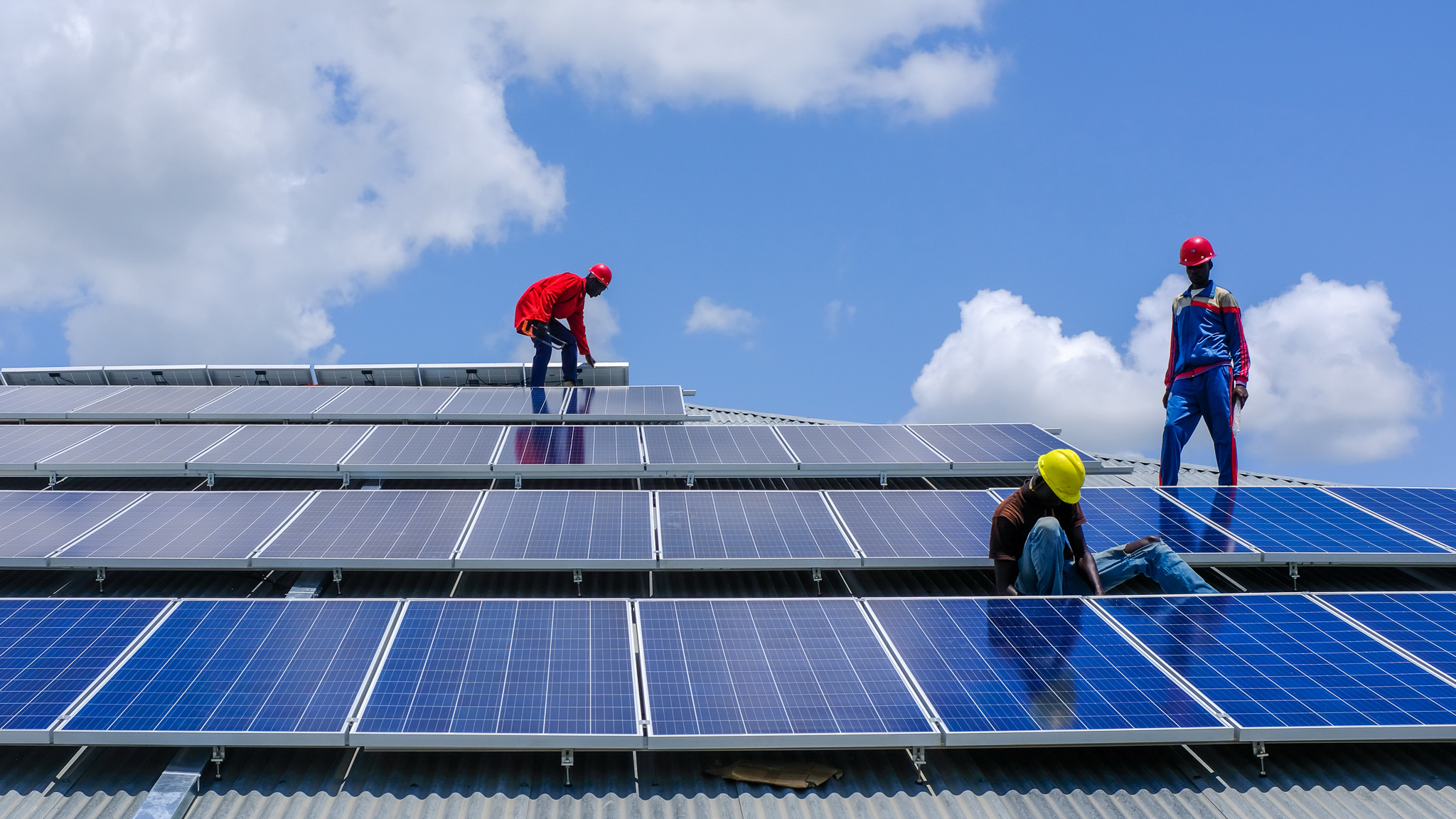In this vibrant, outdoor, landscape photograph, three African American workers are diligently installing solar panels under a bright blue sky dotted with fluffy white clouds. The image, taken from a slightly upward perspective, showcases four ascending rows of blue rectangular solar panels with white grids, prominently filling the frame. A glimpse of a gray roof is visible around the edges.

In the foreground, a worker is seated between the first and second rows of solar panels. He is wearing blue jeans with a rip at the knee, a short-sleeved brown T-shirt, and a yellow safety helmet. His focus is directed toward the solar panel in front of him. Standing to his right, another worker clad in a red hard hat and a matching blue and red track suit observes him attentively.

Above, near the fourth and highest row of panels, a third worker is bent over, engaged in installation tasks. This worker is distinguished by his billowy red long-sleeved jacket, dark pants, and a red safety helmet. The cloud-speckled azure sky occupies the upper half of the photograph, emphasizing the clear, sunny conditions under which this critical work is taking place.